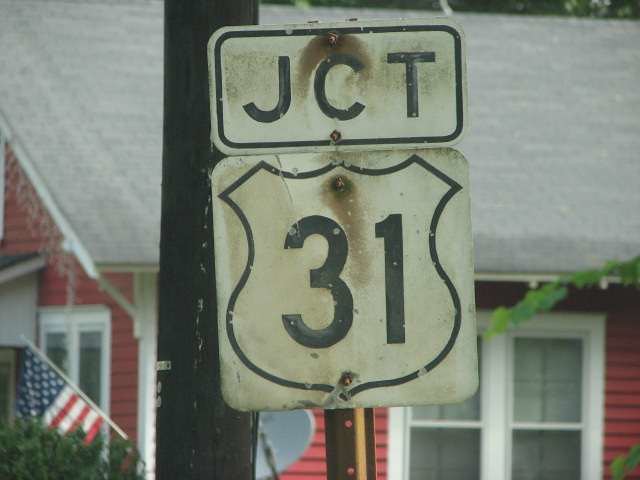This outdoor photograph features a two-story house as the background, showcasing its architectural details. The house has a roof covered with gray shingles, occupying approximately half of the image's backdrop. Its dark wood siding provides a striking contrast to the roof, while an American flag hangs proudly from the facade. The house also features two white-framed double windows, adding to its character.

Prominently in the foreground stands a utility pole, which appears dirty and weathered. Directly in front of this pole is the main focus of the photograph: a duo of street signs mounted on a rusty metal bracket. The top sign is a white rectangle with "JCT" written in black font, indicating a junction. Below it, a square sign featuring a shield bears the number "31," marking a specific route or highway. The signs and utility pole create an interesting juxtaposition against the residential backdrop.